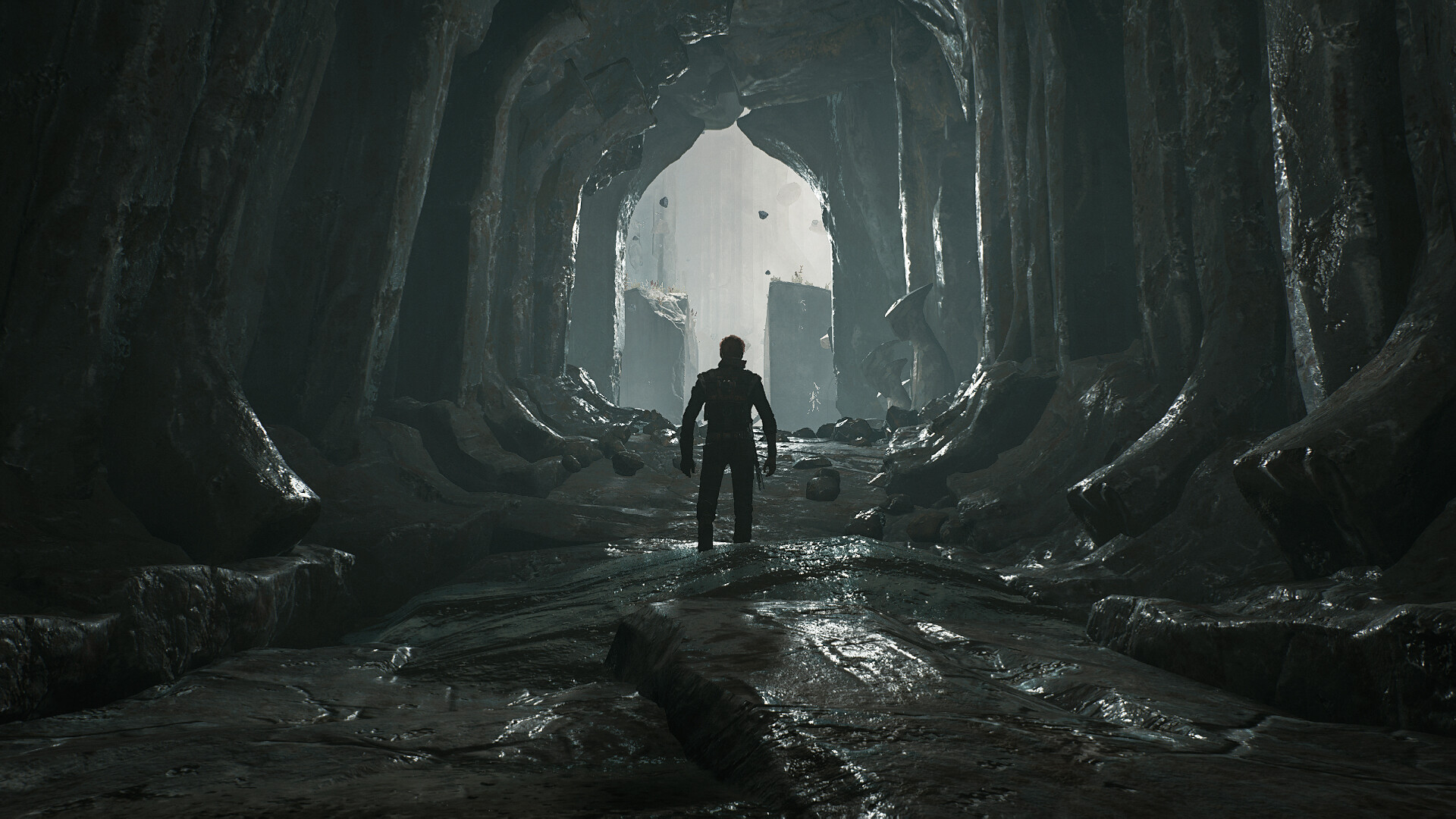A computer-generated image depicts a futuristic character, possibly a space explorer, standing in a moisture-laden stone cave. The character is dressed in a detailed spacesuit, sans helmet, with intricate patterns and high-tech elements visible on the suit and jacket. The cave, adorned with glistening rocks, features a damp environment that reflects light making the stones shimmer. A winding path leads through the cave, the ceiling arching into a semi-dome, guiding the eye towards an opening bathed in bright light. In the distance, two rectangular structures emerge through the illuminated exit, hinting at an advanced world beyond the cave's mouth.